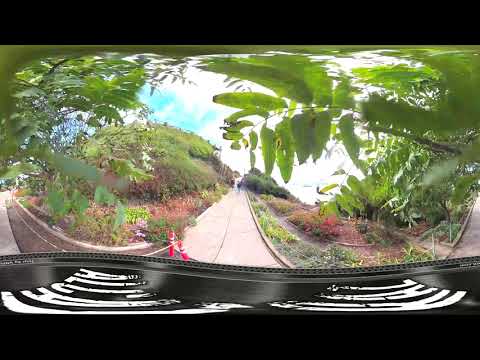The image portrays a vividly distorted view of a garden path or road, possibly seen from a warped camera lens or through a car windscreen. The pathway, constructed with gray cement and flanked by low walls, extends into the distance where indistinct figures are visible walking. This area is enveloped in dense foliage, with an abundance of greenery, trees, and colorful flowers on both sides, visually blocking much of the vibrant blue and white sky. The scene is accented by orange, black, and white cones placed near the front of the image. The right side of the path features lush shrubberies and grass, while the left side bursts with colorful bushes and flowering plants. The large tree in the foreground stands close, providing an intricate view of its lush leaves. Despite the distortion and warping effect, the vivid blooms and blossoming trees suggest a warm and inviting garden atmosphere, rich with the scents and colors of the season.